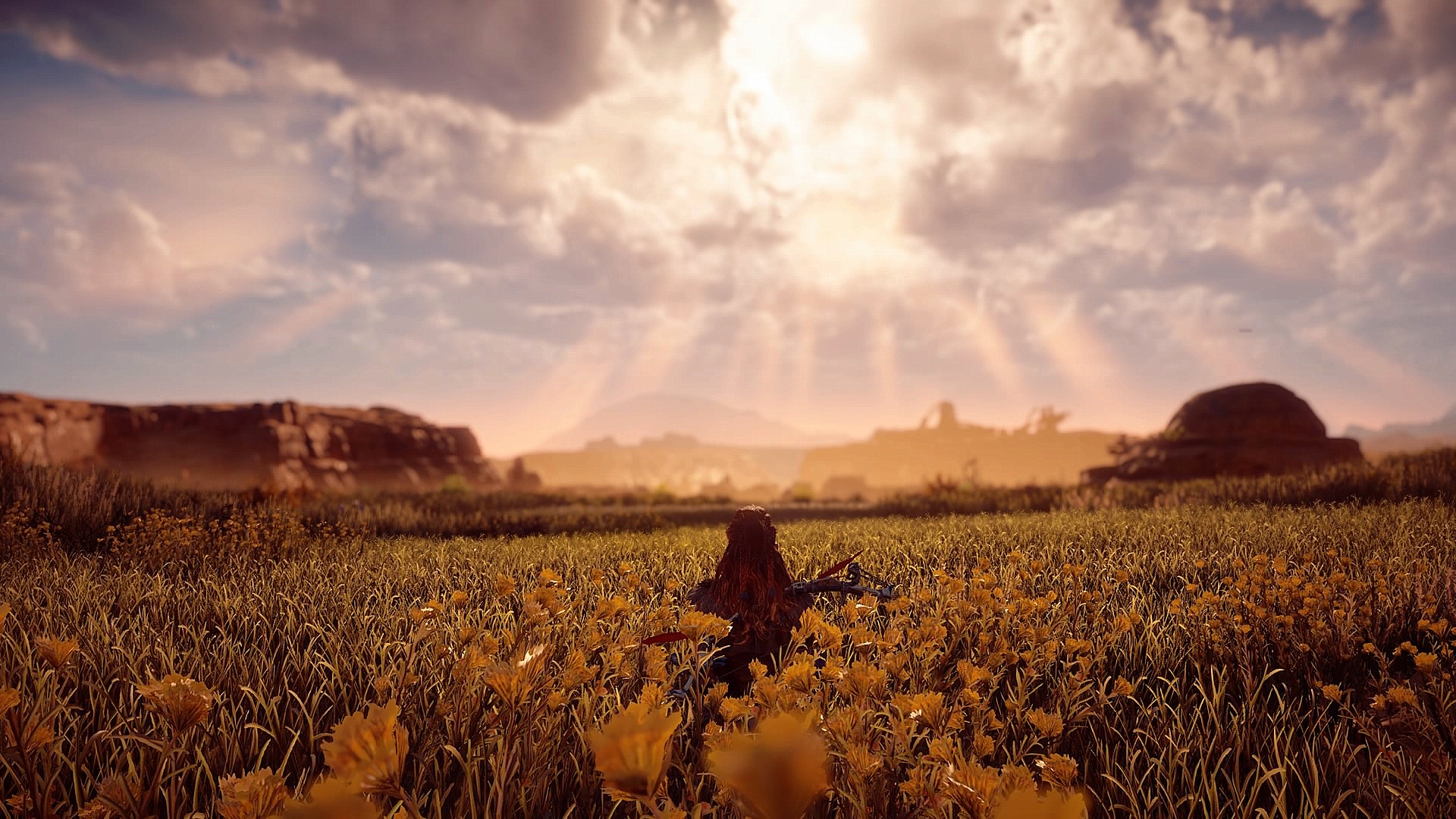A vibrant meadow stretches across the foreground, adorned with an abundance of yellow flowers interspersed with lush green grass. Dominating the center of the area is a sizable tree stump, weathered and brown, adding a rustic element to the scene. In the top left corner, a rugged cliff rises, composed of large, reddish-brown rocks and stones that contrast starkly with the greenery below. The middle section, extending to the top right, reveals more elevated terrain, resembling hills or cliffs, sporadically dotted with various objects. Adjacent to this, a prominent, rounded rock formation of the same reddish-brown hue creates a point of interest on the right side of the image. Above, a brilliant blue sky is punctuated by fluffy white clouds, with a radiant beam of sunlight piercing through the middle, casting warm sun rays across the upper portion of the landscape.